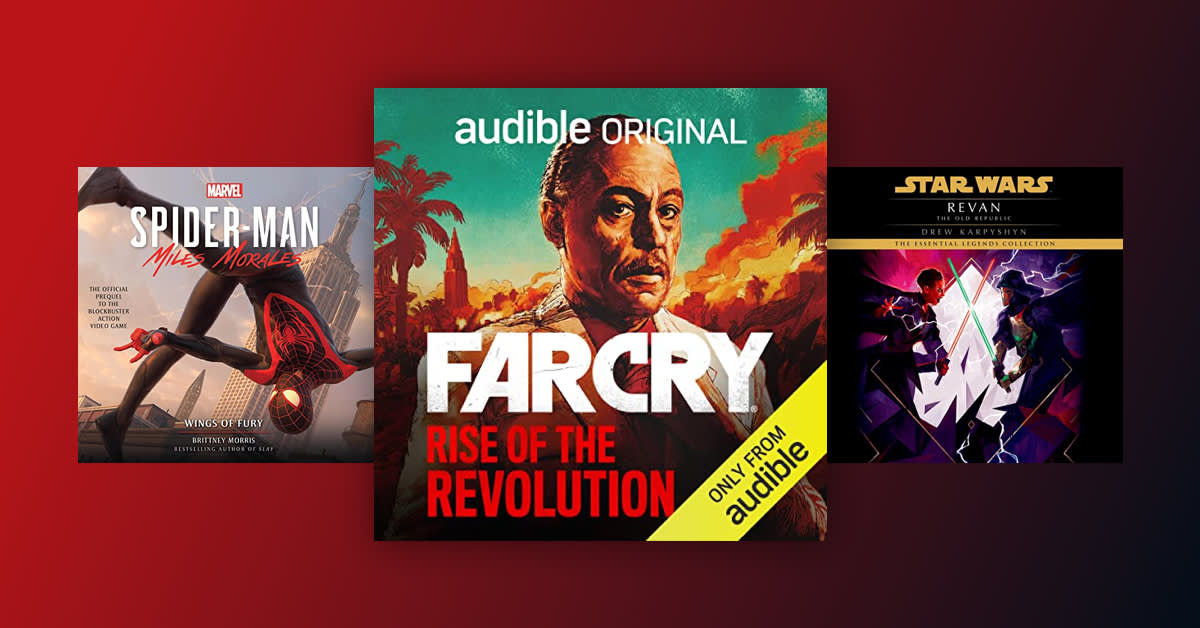The image features three square movie covers arranged side by side against a rectangular background that gradually ombres from bright red on the left to almost black on the right. The covers, which belong to Spider-Man, Far Cry: Rise of the Revolution, and Star Wars: Revan, suggest that this could be an interface where one might click to watch the respective movies.

On the left, the cover displays **Spider-Man, Miles Morales: Wings of Fury**, featuring Spider-Man in a black suit, flipping upside down against a backdrop of high-rise buildings. The center cover is for **Audible Original's Far Cry: Rise of the Revolution**. It shows an illustrated, balding man with reddish features and fires raging behind him. The text "Far Cry" is in white, while "Rise of the Revolution" is in red, and a yellow banner at the bottom right corner states, "Only from Audible" in black. On the right, the cover highlights **Star Wars: Revan**, depicting a duel between a Darth Vader-like figure and another character, both crossing sabers.

The distinctive square icons and the vibrant ombre background enhance the visual appeal, making the image striking and immersive.